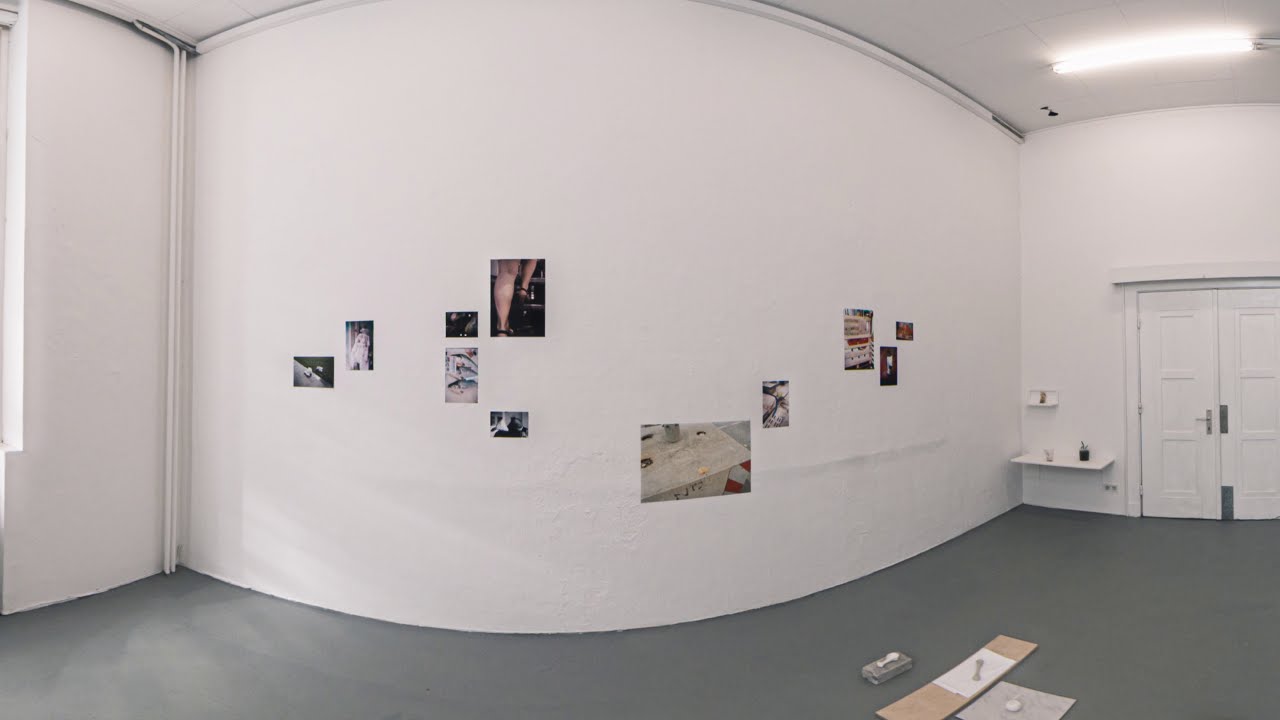In this image, we see a wide-angle view of a spacious, almost empty indoor room. The room features gray floors, which could be either carpeted or hard, and bare white walls. The walls are adorned with several pictures: a large picture in the center and smaller ones scattered on either side, depicting various scenes, including a person standing and what looks like women's calves walking up black stairs. On the far wall, there's a white shelf holding small potted plants with black pots and green foliage. The wall with the pictures seems to curve slightly, which may be a result of the wide-angle lens effect. To the left, there's a large window, and to the right, a white door with silver handles. In the center of the floor, there are a few unidentifiable wooden objects. The lighting suggests it is daytime, contributing to the bright, inviting ambiance of the room. The colors visible in the image include white, black, tan, gray, yellow, and red. There is no text visible anywhere in the image.